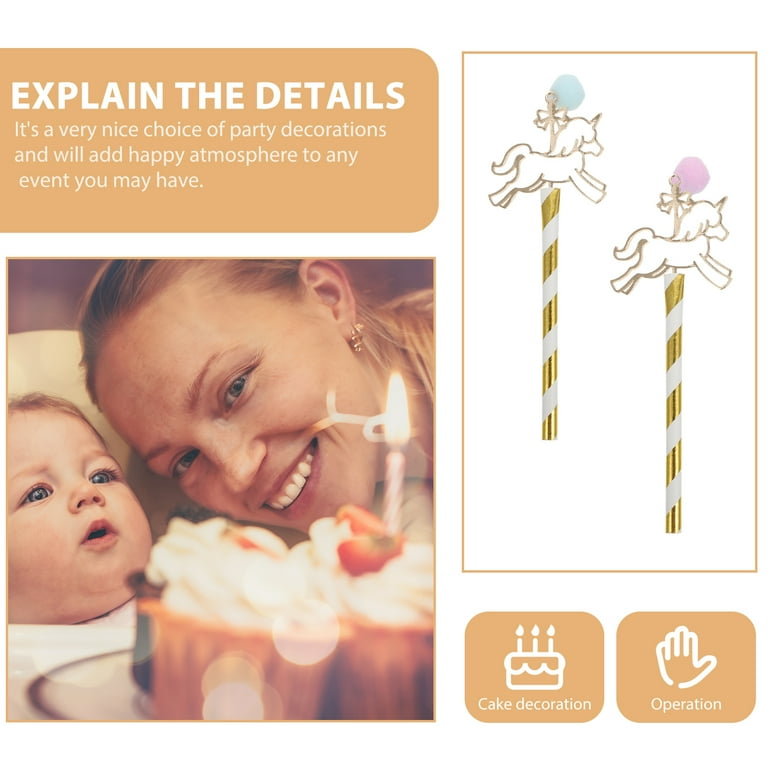This image is an advertisement for birthday cake decoration candles. The image features a white background with accents of gold and a matte golden ivory color. On the lower left, there's a photograph of a young blonde Caucasian woman posing with her young baby, both of them smiling and focusing intently on a plate of cupcakes with one of the lit candles. The baby has an open mouth, captivated by the light of the candle.

The upper right section of the image displays two cake candles with a gold-and-white striped design, each topped with a golden unicorn outline and a pom-pom. The left candle has a light blue pom-pom, while the right one has a light pink pom-pom. 

In the upper left corner, golden ivory squares provide details about the product, labeling it as a cake decoration and emphasizing how it will add a happy atmosphere to any event. The text "explain the details" is featured prominently, guiding the viewer's attention to the product's features. The overall composition effectively showcases the festive and whimsical elements of the birthday candles, making them an attractive choice for party decorations.